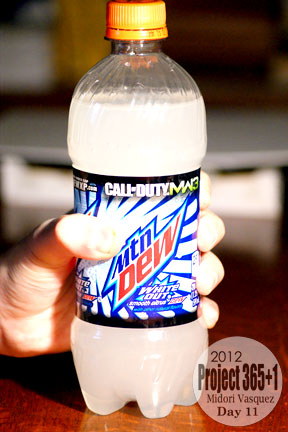In this image, a young Caucasian person is holding a clear, 20-ounce Mountain Dew bottle with their left hand, resting it on a brown wooden table. The bottle, featuring an orange cap, is filled with an opaque white soda labeled as Mountain Dew White Out. The label design is primarily black with vibrant white and blue accents, and prominently displays a Call of Duty MW3 promotion, suggesting it targets a younger audience. The lower right-hand side of the image showcases a round disc that states "2012 Project 365 Plus One, Midori Vasquez, Day 11," adding a unique context to the photograph. The background appears nondescript with a hint of a silvery object in view.